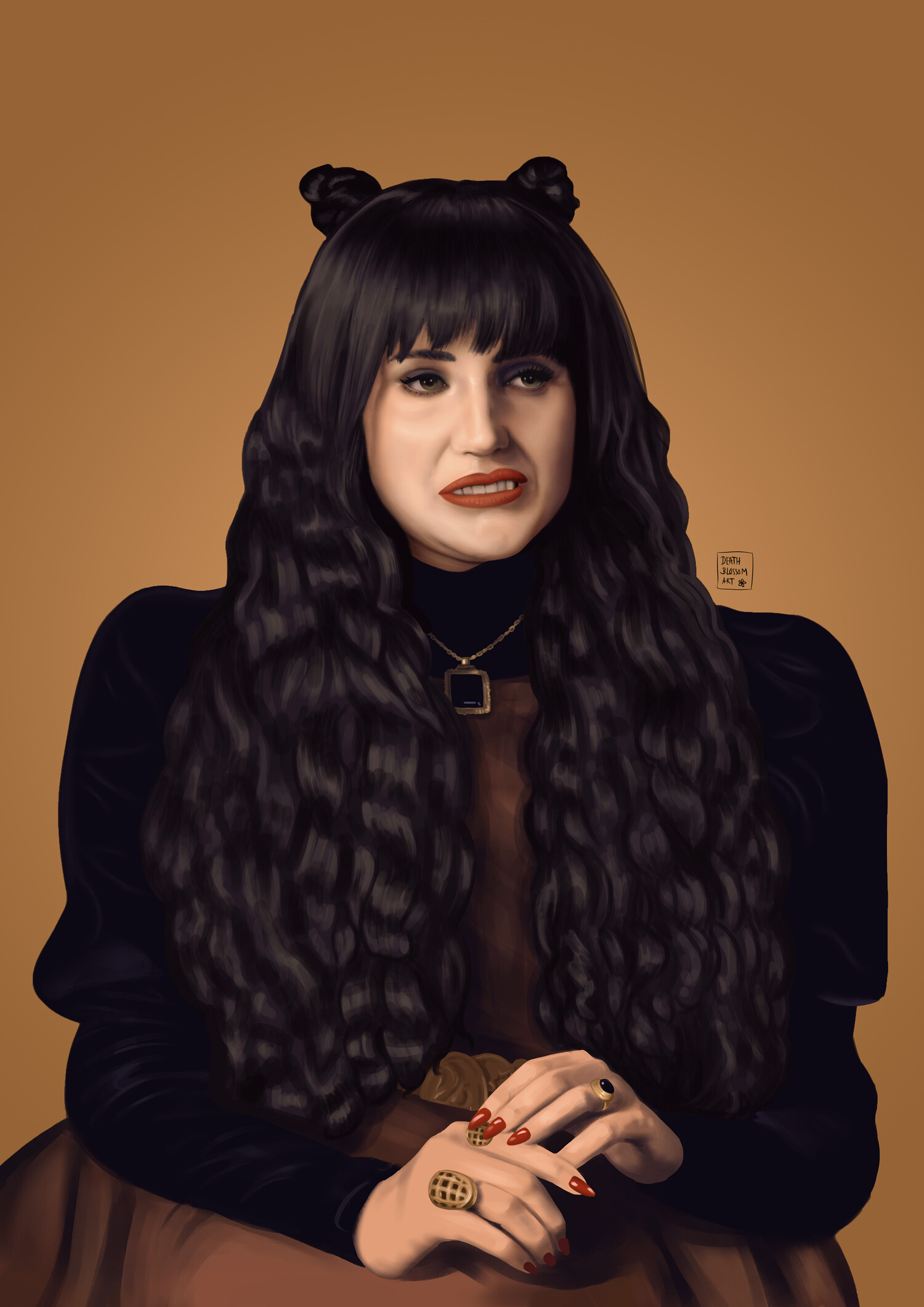This detailed artwork depicts a character, resembling Nadia from the television series "What We Do in the Shadows," seated in front of a brown backdrop. She is positioned facing the viewer, with her gaze slightly averted to her left. Her most striking feature is her long, flowing black hair, which cascades down to her waist with curls at the bottom. Part of her hair is styled into two small buns on the crown of her head, resembling ears or knobs. She has bangs that frame her face. Her expression is complex, a combination of a half-smile and a look of slight disgust or a sneer, accentuated by her red lipstick.

She wears a striking ensemble consisting of a black long-sleeve jacket over a brown poofy dress that flares out at the bottom. A gold necklace with a black onyx square pendant adorns her neck. Her hands, decorated with red nail polish, are placed on her lap, revealing two interesting rings—a small black ring on her left hand and a larger golden oval ring on her right. Additionally, a belt with circular gold discs is partially visible beneath her hair. The image has the appearance of a digital artwork, capturing the detailed elements of her attire and expression vividly.